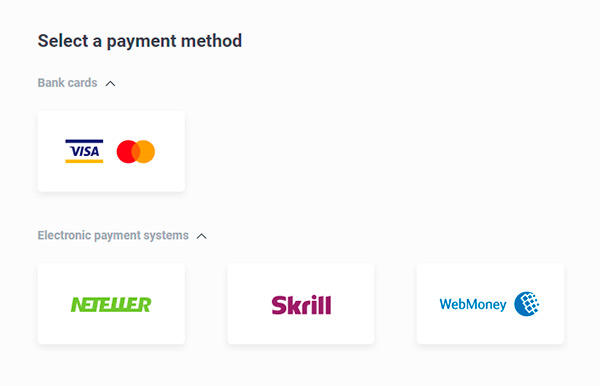The image depicts a payment screen interface, likely viewed on a digital device such as a smartphone, tablet, laptop, or desktop. The user is prompted to select a preferred payment method. Options for payment include traditional bank cards with support specifically for Visa and MasterCard. Additionally, there are electronic payment options available, displayed prominently with their respective icons. 

To the right of the Visa and MasterCard logos, the digital wallet options include:
1. NetTeller - indicated by its distinct icon.
2. Skrill - positioned immediately to the right of the NetTeller icon.
3. WebMoney - displayed next to the Skrill icon.

These digital wallets offer alternative methods for completing the transaction. Overall, the screenshot illustrates that users can choose between conventional bank cards (Visa or MasterCard) or digital wallets such as NetTeller, Skrill, and WebMoney, providing flexibility in how they wish to pay for goods or services on the website.